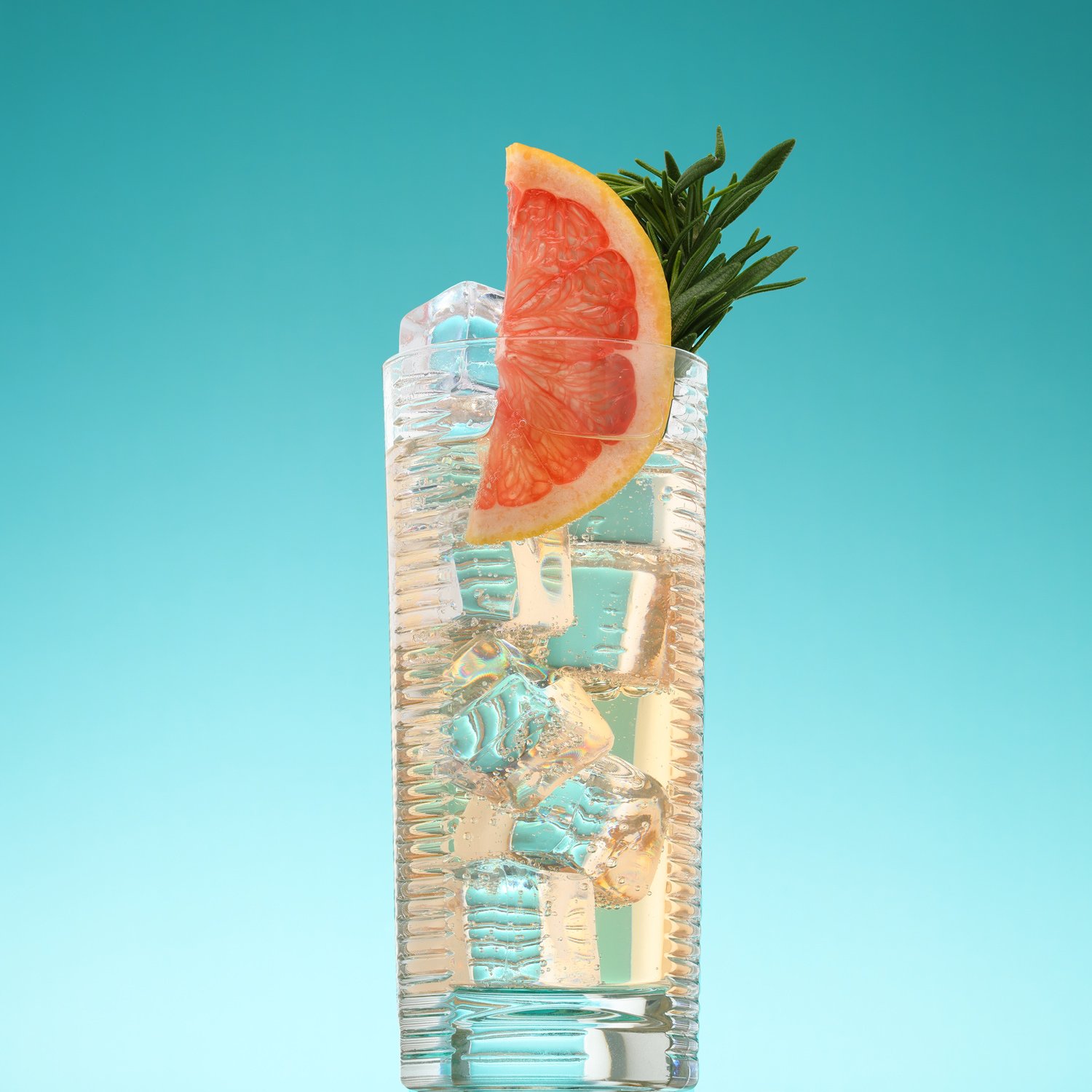The image is a striking photo-realistic shot centered on a tall, clear glass filled with a light gold, transparent beverage, possibly carbonated and slightly alcoholic. The glass is adorned with ridges or rivets that provide a textured grip, and it features a thick, clear base that subtly warps the light, adding to the visual interest. Several clear square ice cubes are stacked nearly to the rim, with one protruding slightly above it. Nestled among the ice is a fresh sprig of dark green mint or thyme, adding a touch of vibrant greenery. On the right side of the glass, a thin slice of grapefruit, showcasing its red, juicy flesh and yellow rind, is inserted into the liquid. The background features a teal gradient that shifts from a darker shade at the top to a lighter hue towards the bottom, creating a refreshing and serene ambiance that complements the cool, crisp appearance of the drink.